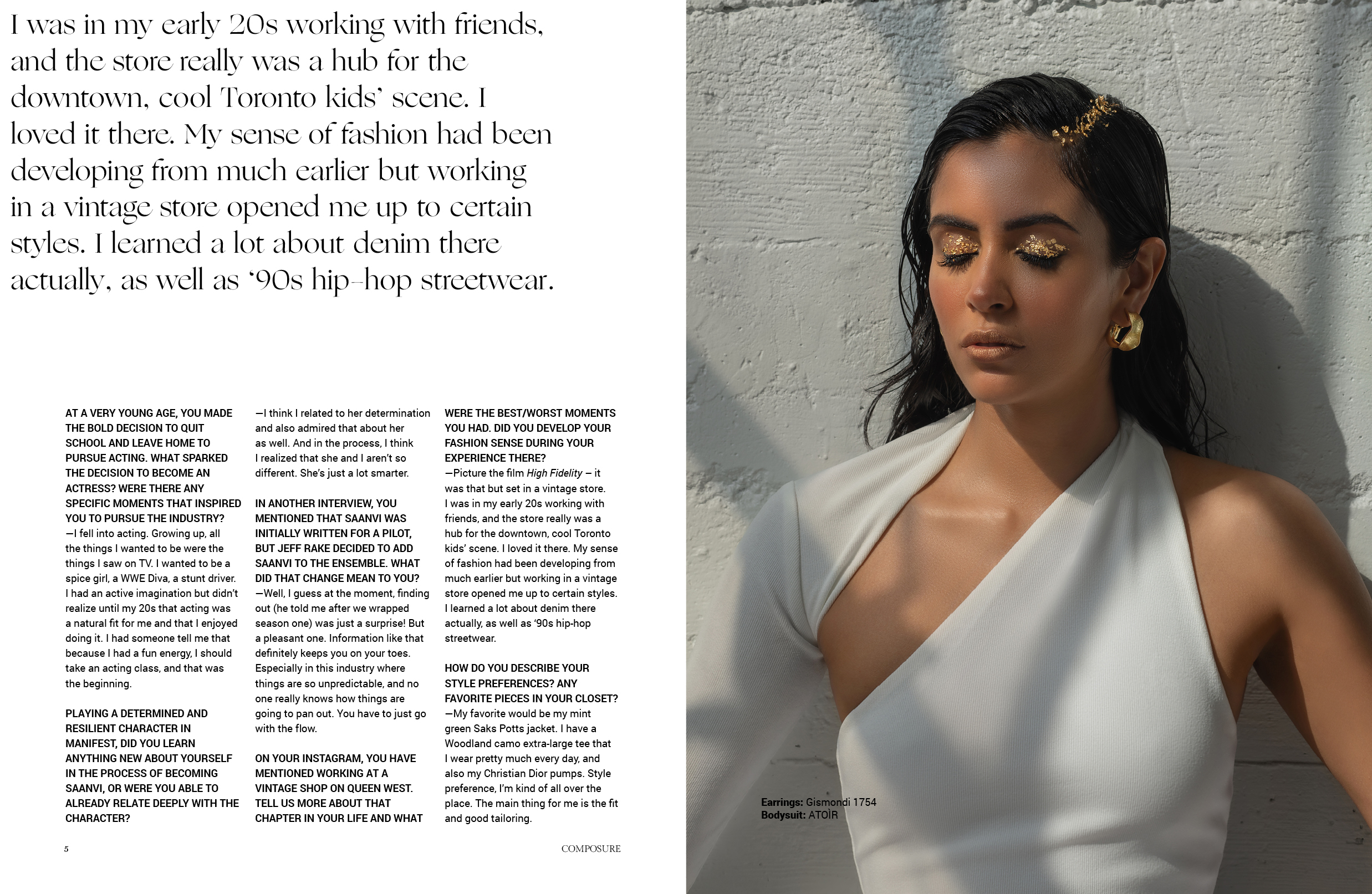This full-color image, presented without a border, is essentially square in shape. The background features a mix of a gray stone or brick wall on one side, contrasting sharply with the white of the screen on the other. The right half of the image is dominated by a photograph of a young woman, possibly of Spanish or Middle Eastern descent, with mid-toned skin and dark black hair that cascades loosely behind her back. Her eyes are closed, showcasing bright gold eyeshadow and black lashes, enhancing her striking features. She wears a unique white dress with an off-shoulder design on her left side and a full shoulder and sleeve on her right, further detailed with a wrap-around element at the neck. Completing her elegant look are gold earrings and a gold beret, as well as a touch of gold glitter at her hairline. The left side of the image is filled with text, likely an excerpt from a journal, blog, or magazine article named "Composure." This text narrates the author’s experience in their early twenties, working in a vintage store that was a vibrant hub for the cool youth scene in downtown Toronto. The narrative highlights the author’s evolving fashion sense and the influence of working with vintage styles, particularly noting a newfound interest in denim and 90s hip-hop sportswear.